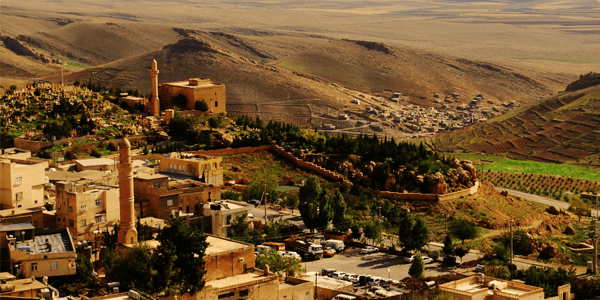This aerial photograph features a town perched on a hillside in a fairly barren region, likely a Middle Eastern area based on the architectural elements. The town is composed predominantly of tan or sand-colored buildings, closely packed together. In the foreground, there's a parking lot and various vehicles, suggesting a modern setting. A small stone fence encircles part of the hill, where there are trees and a rocky formation. Notable are two towers that rise above the other structures, reminiscent of those found in Middle Eastern architecture. The background reveals rolling, brown hills with sparse vegetation, devoid of buildings or human activity. Further down into the valley, one can find additional sporadic buildings and potentially some cultivated fields. The overall scene blends the greens of trees and crops with the browns of the earth and buildings, creating a cohesive natural and urban landscape.